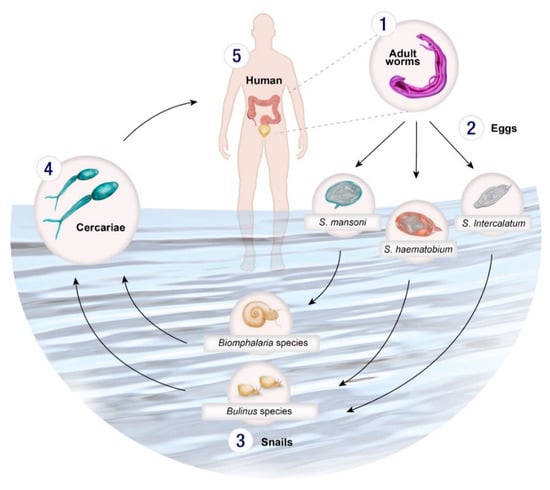The illustration depicts the lifecycle of a parasitic worm, showing its progression through various stages and hosts. Starting with an adult worm labeled as number one, the image then transitions through several types of eggs (S. mansoni, S. haematobium, S. intercalatum) marked as number two. These eggs transform into larvae species, which include references to Biomphalaria and Bulinus snails, depicted at stage three. The lifecycle continues with the cercariae stage, labeled as number four, which are organisms resembling small, worm-like shapes. Finally, it concludes with a human host at step five, shown standing in blue-colored water, indicating the transmission vector. Black arrows trace the sequence of stages in a circular pattern, emphasizing the continuous nature of the parasitic cycle. The human figure, peach-colored and outlined, highlights the end point of the parasite's journey as it infects the individual’s body, with a focus on the intestines. The detailed arrow and number system visually clarify the parasitic path from worm to human host.